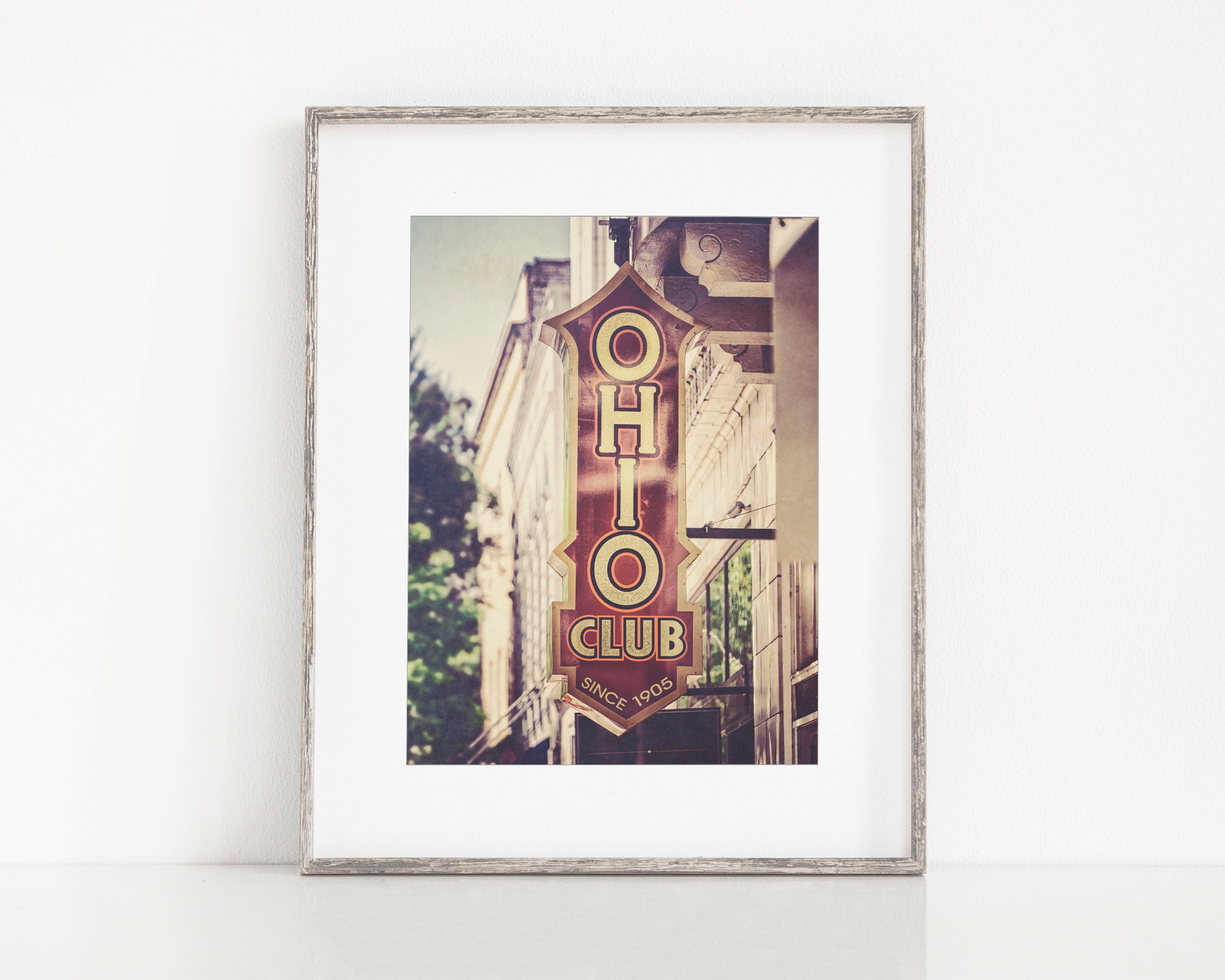The image features a photograph of a poster displayed in a light gray, natural wood-look frame with a large white border. The poster itself is a photograph of an arrow-shaped club sign with yellow text reading "Ohio Club since 1905," hanging off a black pole from the side of a building. The building, tan-colored and old-fashioned, occupies the right side of the image, while trees are visible on the left. The frame and poster are placed on a flat, glossy white surface, leaning against a flat white wall. The overall setting and composition suggest that this photograph is likely intended for an online listing to sell the poster.